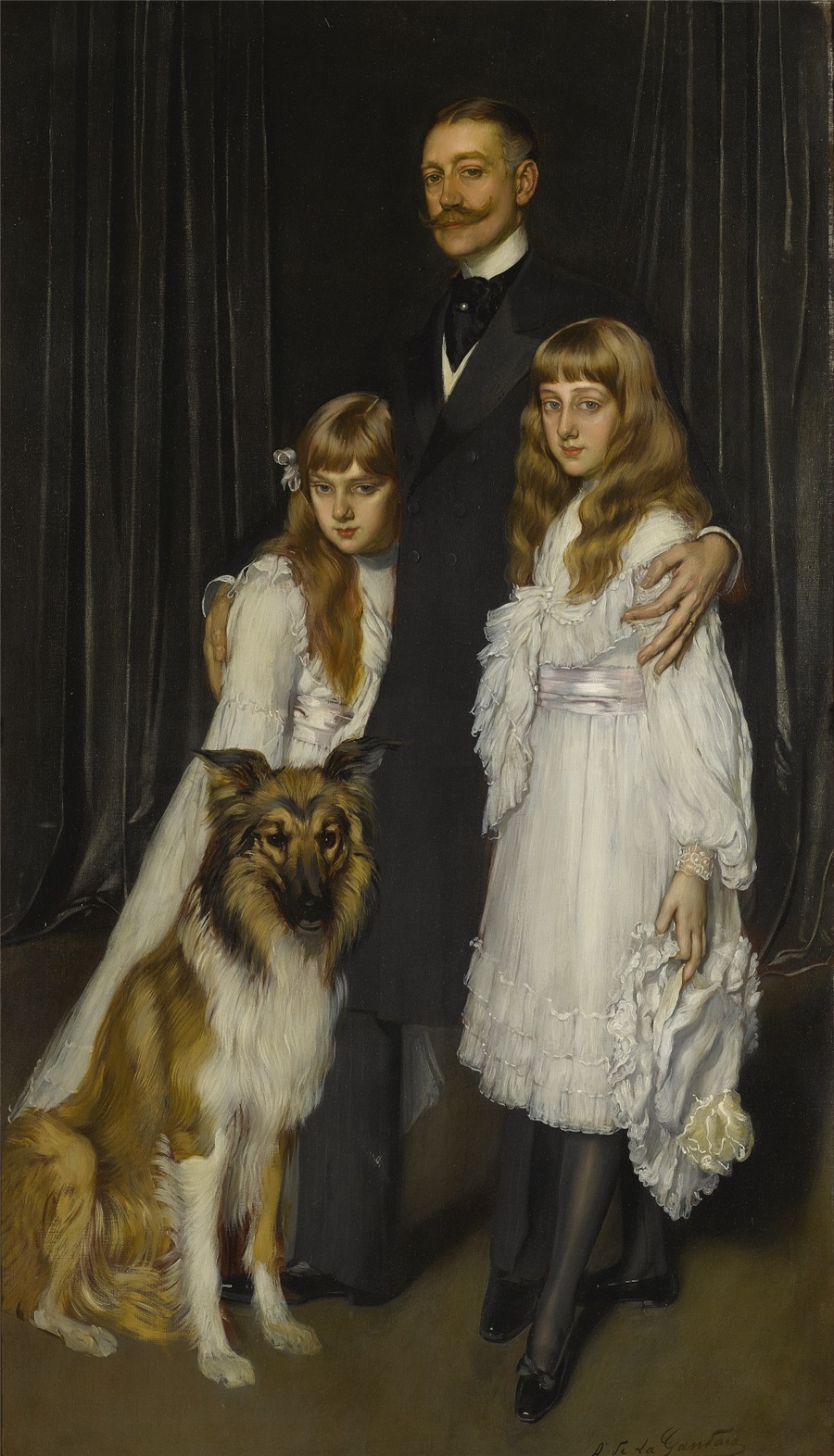A formal oil painting features a tall, distinguished man with a receding hairline, brown hair graying at the sides, and a wide handlebar mustache. He has brown eyes and is dressed in an antique black suit with a white shirt underneath, a tall white collar, and a brown bow tie. The man is holding two young girls, each standing on either side of him with his hands resting on their shoulders. The girls, who appear to be his daughters, are dressed in matching elegant calf-length white dresses, hinting at the late 1800s to early 1900s fashion. Both girls have long brown hair, with one sporting short bangs and the other possibly a blue or gray bow. The girl on the right, who seems to be about 12 or 13 years old, wears black stockings and black shoes, while the girl on the left is slightly younger, possibly around 10 or 11. In front of the family is a large German Shepherd dog sitting and staring directly at the viewer. The setting is indoors with a large black drape or curtain with streaks of gray in the background, enhancing the formal and affluent atmosphere of the portrait. The composition clearly excludes a mother figure, focusing instead on the father with his two daughters and their faithful dog.